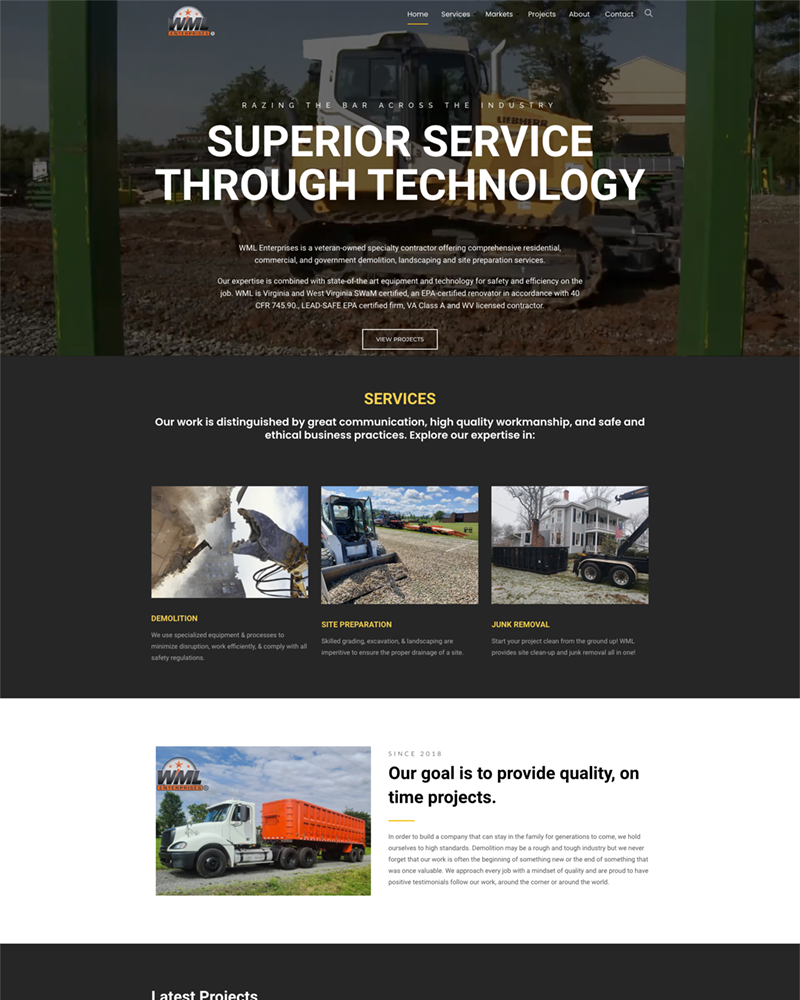Caption:

"WML Enterprises: Raising the Bar Across the Industry. Veteran-owned and specializing in comprehensive residential, commercial, governmental, landscaping, and site preparation services, WML utilizes state-of-the-art equipment and technology to ensure safety and efficiency. EPA certified and West Virginia WAM certified, WML offers superior service through their expertise. EPA certified renovators and VA Class A and WB licensed contractors, WML is dedicated to excellence in all their projects. Featuring a powerful tractor in action, modifying glass and working with dirt, this image showcases the precision and dedication of WML's specialty contracting services."